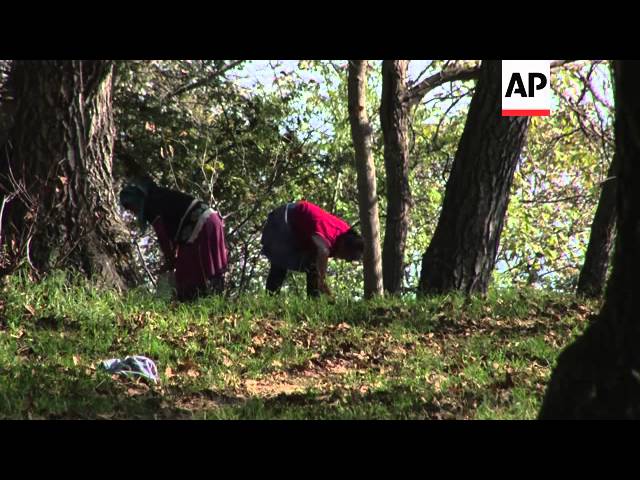A photograph captures two individuals amidst a verdant forest scene, characterized by lush green grass, abundant leaves, and towering trees with coarse bark. The sky is a very light blue, providing a serene backdrop. At the center-left of the image, the two individuals are bending over as if picking up items from the forest floor, likely walnuts, given the context. The person on the right, whose profile is visible, wears a purplish skirt paired with a darker shirt, while the individual on the left dons a red top and dark pants. A brown horse stands nearby, hinting that they may have arrived on horseback. The scene is framed with a black border on the top and bottom, and in the upper right corner, there is a white square with the letters "AP" and a small red rectangle underneath it. Sunlight filters through the canopies, illuminating the activity below as the villagers engage in the seasonal walnut harvest near the village of Arslanbob in southern Kyrgyzstan.